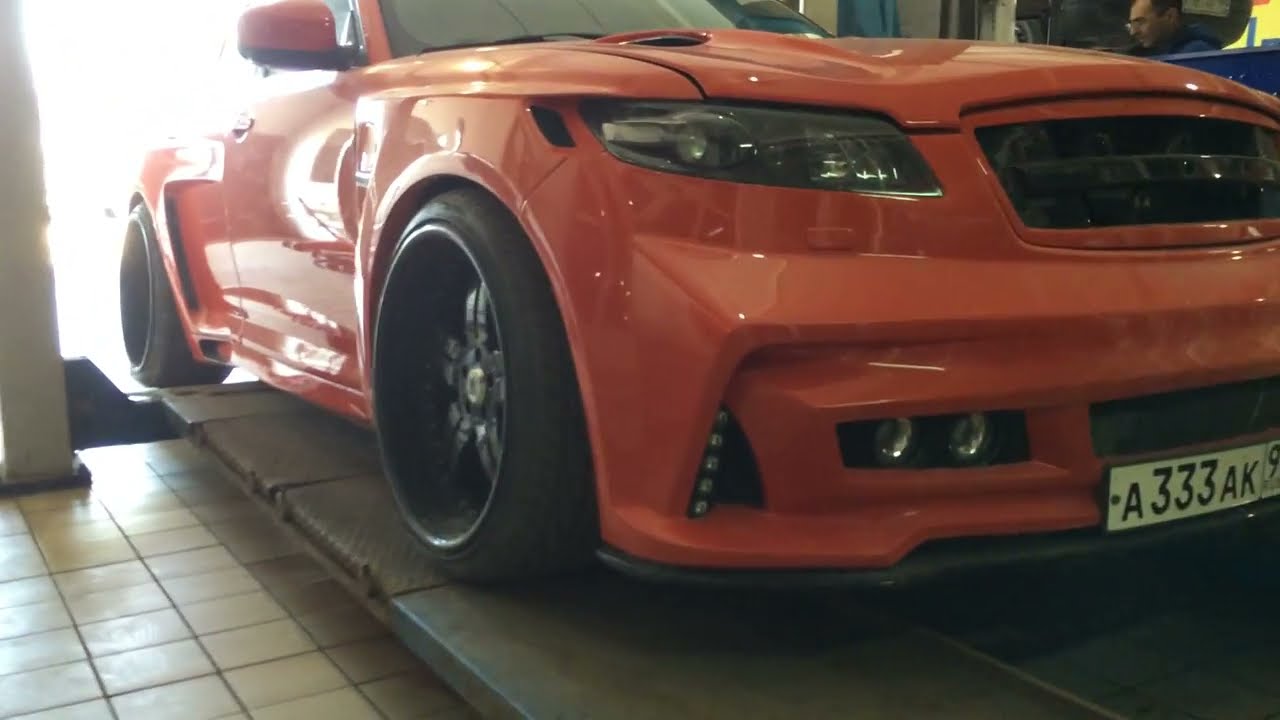The photograph captures the front end of a newer reddish-orange car, which appears to be a combination of red and orange hues. The car is partially elevated on concrete ramps situated on a white checked tile floor, indicative of an automotive repair shop setting. A visible white license plate with the number A333-AK97, in black letters, is mounted horizontally across the lower front bumper. The car features a distinctive body kit and large tires with black deep-dish rims. To the right of the car, there's a blue counter and a partially visible man dressed in black trousers and black work shoes, suggesting the presence of a mechanic. The background includes blurred elements in blue and red, and other vague automotive equipment, enhancing the impression of a busy repair facility. The image is in landscape orientation and exhibits a photorealistic style.